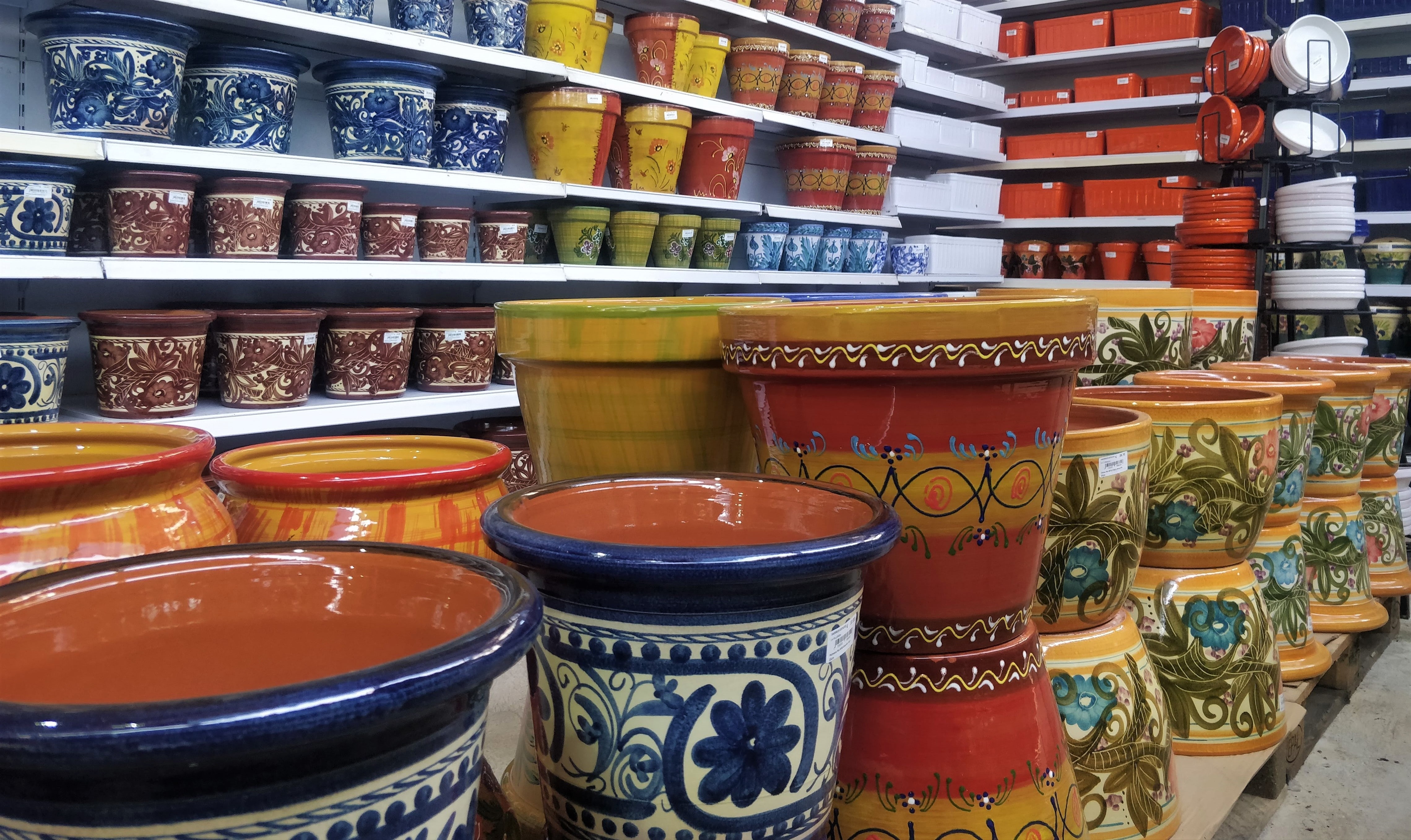A detailed photographic image of an indoor pottery shop showcases a variety of ceramics meticulously arranged throughout the store. In the foreground, a row of large vases or planters dominates the scene, featuring an array of designs. To the left, the first notable vases are blue and white with red linings, followed by a striking orange and brown piece that tapers in the middle, resembling two planters stacked together. Adjacent to these are ten identical vases, characterized by their brown backgrounds adorned with blue and green floral patterns. This row is positioned directly on the floor.

Moving to the background, on the right-hand side of the image, shelves on the wall house an assortment of red boxes. In front of these shelves stands a metal stand displaying white plates on one side and red plates on the other. In the upper left corner, white shelves are visible, displaying smaller vases and planters. These shelves contain a mix of blue and white, red and white, red and brown, light brown, and plain brown ceramics, with the top shelf featuring yellow planters and containers, completing the variety.

The lighting above highlights the ceramics, emphasizing their vibrant colors and intricate designs. The overall atmosphere of the store is one of organized, artistic clutter, inviting viewers to explore the diverse collection of handcrafted pottery.